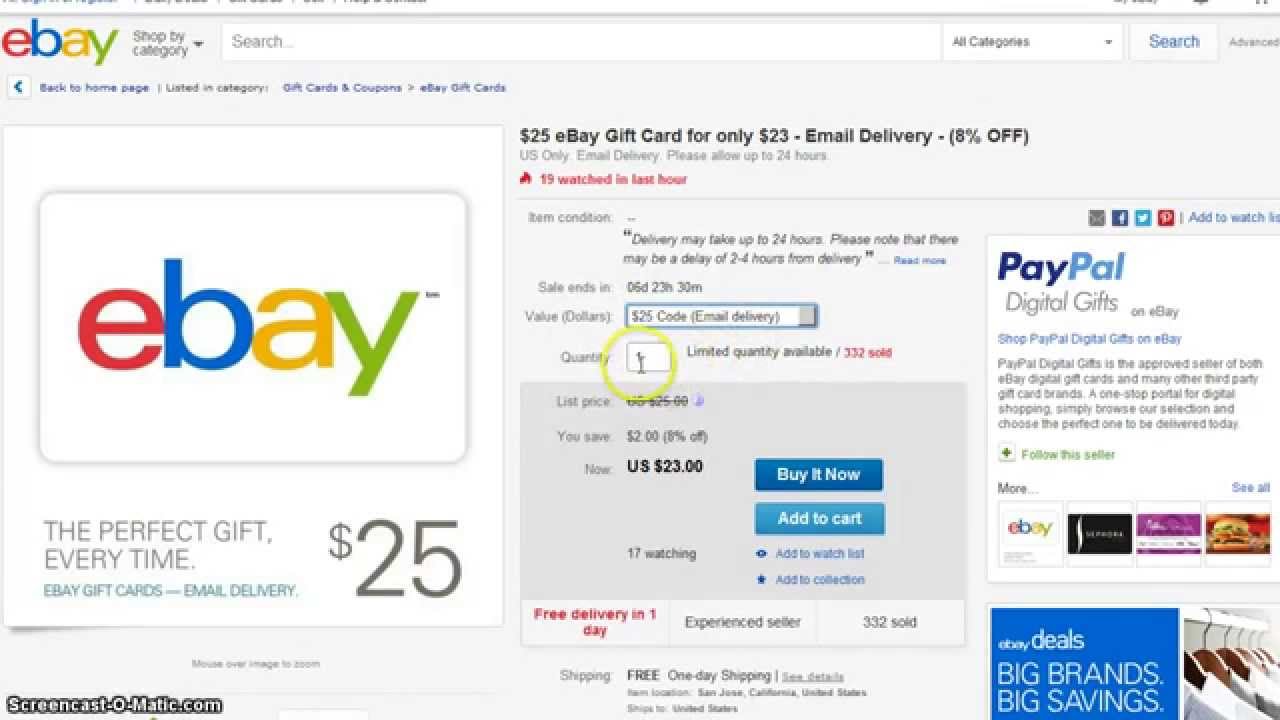The image captures a detailed eBay webpage, prominently displaying a listing for a $25 eBay gift card available for $23 with an 8% discount. In the top left corner, the page includes the "eBay" logo followed by a "Shop by Category" drop-down menu. Next to it, a search bar is positioned with another drop-down filter labeled "All Categories," alongside a search button.

Centered on the page is the highlighted gift card offer, emphasizing the discounted price of $23 for the $25 card, with a note that it is delivered via email. "Email delivery" and "Please allow up to 24 hours" are key details mentioned. The listing also indicates that the card is in demand, with "19 watched in the last hour" displayed.

To the left of the textual description, there is an image of the gift card, illustrating the card with "eBay" printed on it, and beneath it, the phrase "The perfect gift every time $25." Details provided also include "Sales ends in 5 days, 23 hours, and 30 minutes," and specifics such as "Value in dollars: $25" and "Code: Email delivery," with an empty box for "Quantity" highlighted by a yellow circle and a reminder that there is "Limited quantity available" with "332 sold."

Financial details state the savings explicitly: "List price" is crossed out, followed by "You save $2," equivalent to "8% off," resulting in a "New US $23" price. Concluding the listing, there are two action buttons – "Buy It Now" and "Add to Cart" – both in blue with white text.